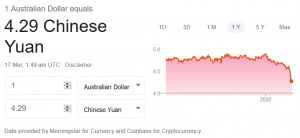This image captures the exchange rate information displayed on a screen, detailing the conversion between one Australian dollar (AUD) and Chinese yuan (CNY). At the top of the screen, it prominently states "One Australian Dollar equals 4.29 Chinese Yuan," with 'Yuan' spelled as Y-U-A-N. Below this, a timestamp indicates "17 Mar, 1:40 AM UTC," accompanied by a disclaimer notation.

The layout features graphical elements representing currency fluctuations; small arrows adjacent to "Australian Dollar" hint at recent currency movement. In a section reminiscent of a chart, "4.29 Chinese Yuan" is reiterated, and there are dropdown menus that allow for the replacement of currencies. Additional information notes that the exchange data is provided by Morningstar for traditional currency and Coinbase for cryptocurrency.

On the right side, a red line graph depicts the exchange rate trend over the past year, illustrating a significant drop from a previous peak to the current value. The visual elements combine to give a comprehensive snapshot of the currency exchange landscape at the specified time.